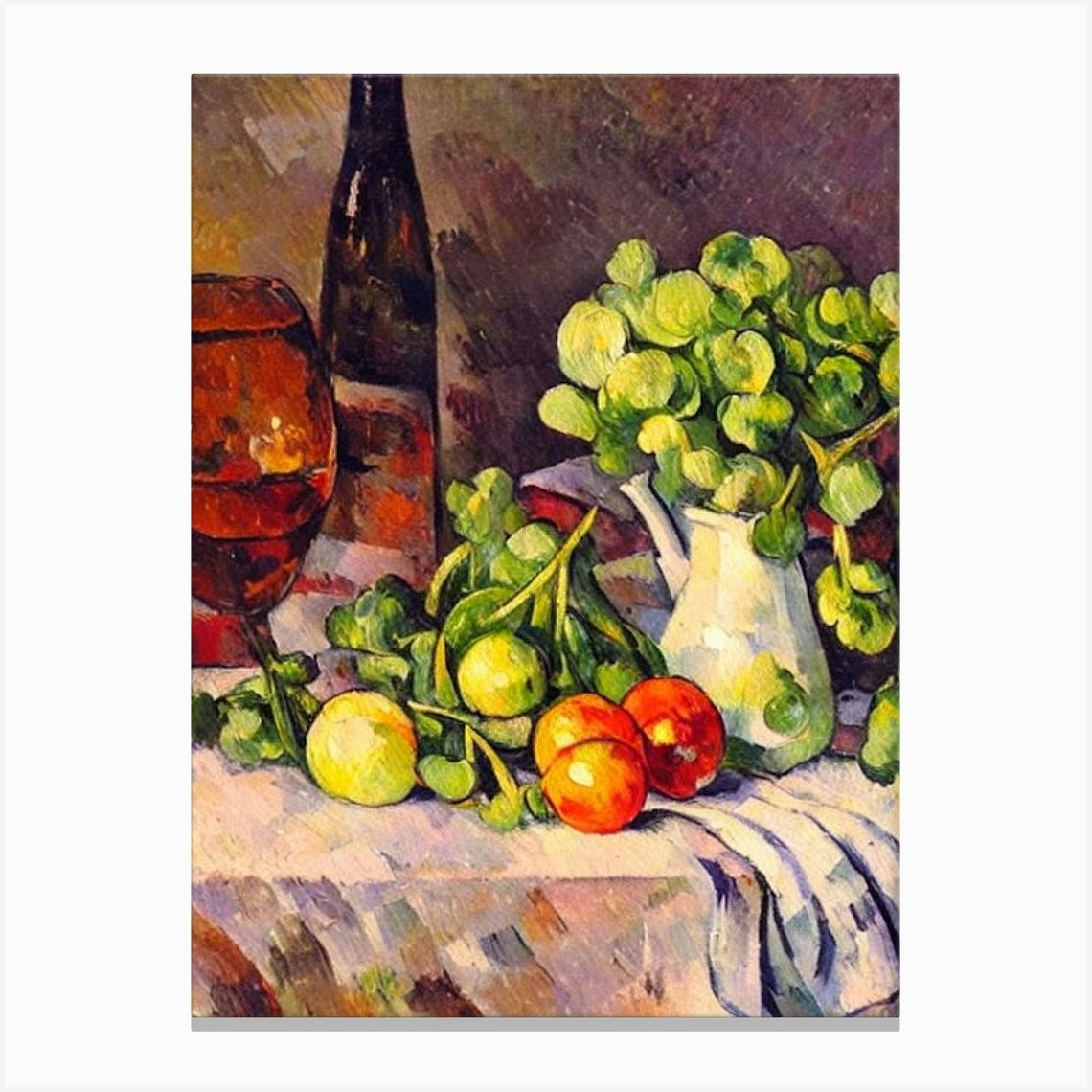This artwork, possibly an oil or acrylic painting, depicts a vibrant and well-balanced still life scene. A table covered with a white cloth forms the setting, with the fabric intriguingly bunched up under a white bottle that appears to have a spout. This bottle, doubling as a vase, overflows with leafy green herbs or plants, adding a lush touch to the composition. 

To the left of the vase, a cluster of fruits can be seen—red and green apples among yellow and green objects, possibly more fruit or nodding leaves from the botanical arrangement. Further left, another vessel, darker and set in the background, creates depth and contrast. Additionally, an amber wine bottle with a white label stands prominently, accompanied by a wine glass half-filled with a liquid in shades of red and burgundy.

The overall color palette is richly diverse, featuring vibrant greens, reds, and shades of gold, balanced by muted tones like brown, black, and gray, with subtle hints of blue. The wall behind the table is a captivating mix of purple and gold hues, enhancing the painting's visual depth and warmth. Each element is meticulously rendered with visible brush strokes, contributing to the tactile quality of the piece. The composition is a harmonious blend of color, proportion, and texture, making it not only pleasing but also compelling in its detail and execution.